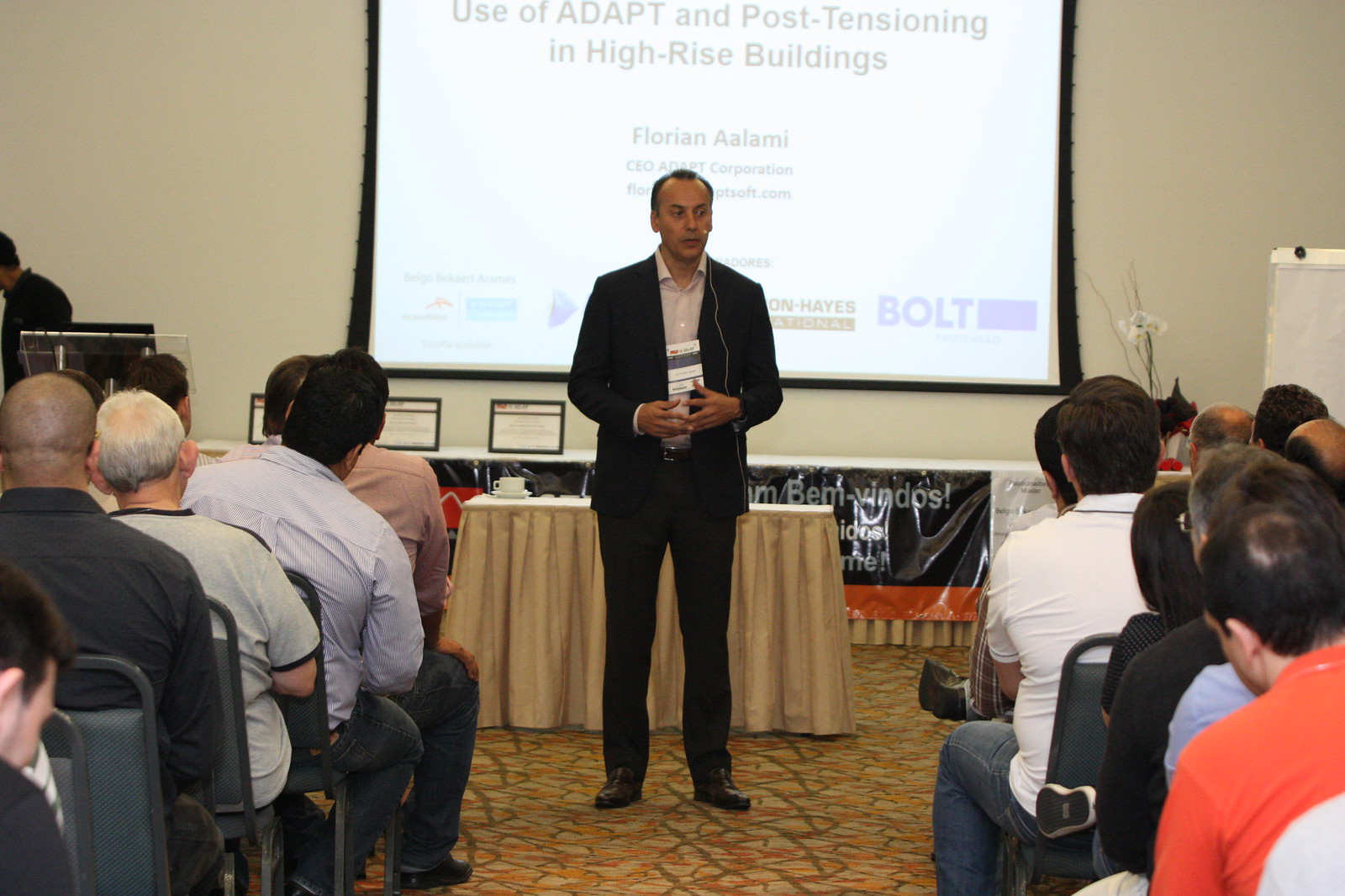The image captures a scene from an audience member's perspective during a presentation in a convention room, likely within a hotel. Central in the image is the presenter, a man named Florian Alamy, standing confidently in a black suit with a light gray, open-collar shirt. He is equipped with a headset microphone and a name tag pinned on his suit. His hands are visible and positioned in front of him as he addresses the audience. The presentation topic, "Use of Adapt and Post-Tensioning in High-Rise Buildings," is displayed clearly on the white projector screen behind him, bordered by a black area and featuring several company logos at the bottom. 

The room features a light brown skirted table directly behind Florian and groups of chairs filled with audience members of varying ages, seated on both sides of the aisle, all attentively facing him. The setting appears somewhat nondescript, typical of large conference spaces used for professional gatherings. The mood in the audience seems to be one of engagement and focus on the technical lecture being presented.